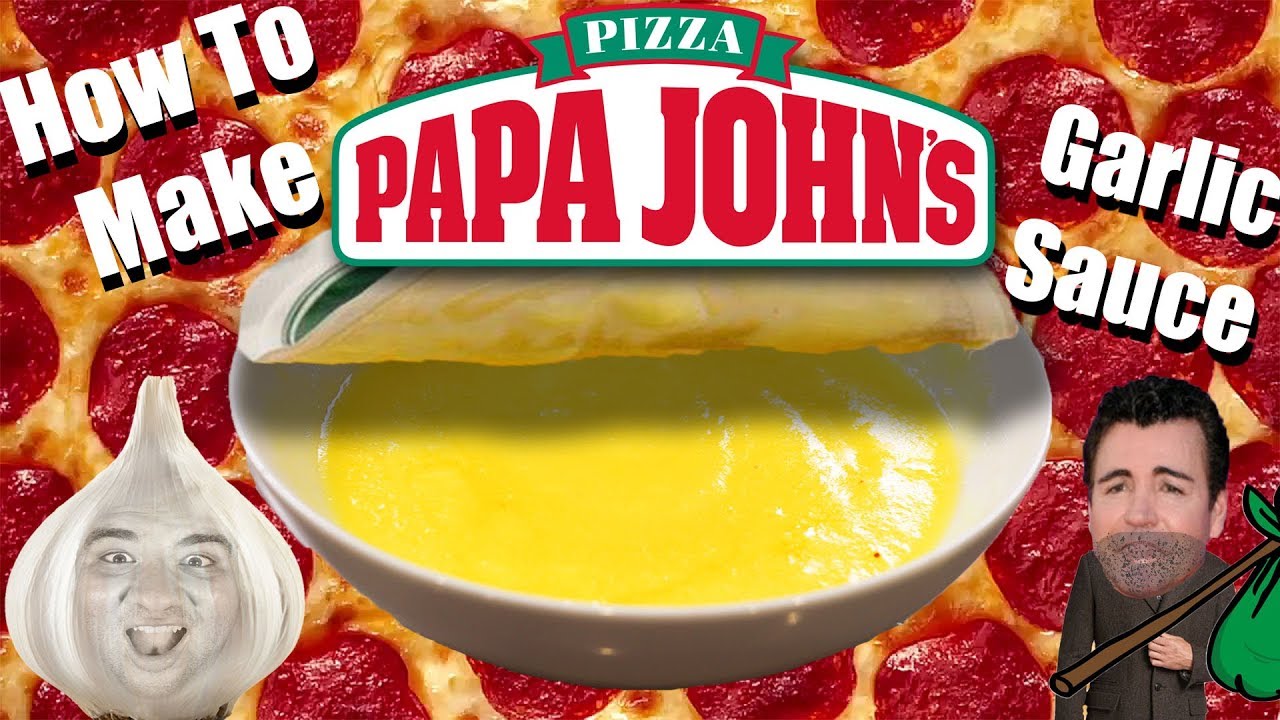The advertisement is a detailed poster for Papa John's, featuring a pepperoni pizza as the entire background. The upper center prominently displays the Papa John's logo in big red letters against a white backdrop, with the word "Pizza" in white letters on a green banner above it. On the upper left corner, it reads "how to make" in white print, and on the upper right corner, it says "garlic sauce," also in white letters. At the center of the image, positioned atop the pizza, is a bowl with a yellow liquid, presumably garlic sauce, with a foil lid partially peeled back. On the lower right is an image of the founder of Papa John's dressed in a green shirt, sporting a scruffy beard, and holding a stick with a green bag tied to it, reminiscent of a hobo's bag. To the lower left, there's a playful depiction of a smiling man inside the bulb of a garlic clove, his mouth wide open in a cheerful expression.